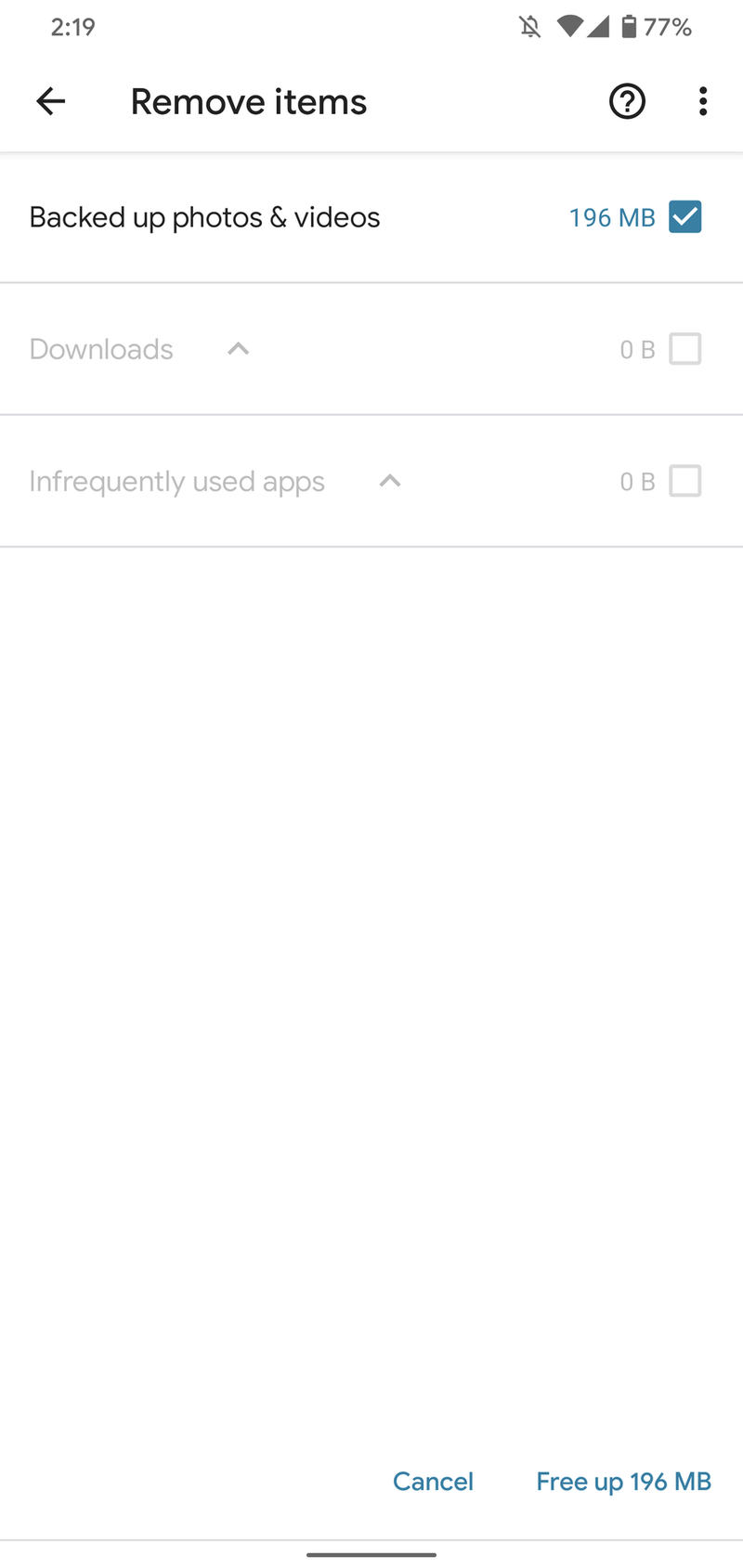**Detailed Descriptive Caption:**

A tall, narrow cell phone screenshot displaying a storage management interface. At the top of the screen, the time is shown as 2:19, alongside icons for volume, Wi-Fi signal, cellular coverage, and battery life, which is at 77%. Below this status bar, a black left-pointing arrow is visible, adjacent to the text "Remove items." A black question mark within a circle and a vertical line of three black dots are located to the right.

Following these navigation elements, the main interface is displayed, starting with a section labeled "Backed up photos and videos, 196 MB," which has a checked box next to it. Under this is a category labeled "Downloads," accompanied by an upward-facing arrow and the size notation "0B," with an unchecked box beside it. Below that, another category titled "Infrequently used apps" presents an upward-facing arrow and the size "0B," with its corresponding box also unchecked. 

At the bottom of the screenshot, options are presented for "Cancel" and "Free up 196 MB." The image strictly contains textual and graphical interface elements, with no visible people, animals, plants, vehicles, or other objects outside of the digital UI components.